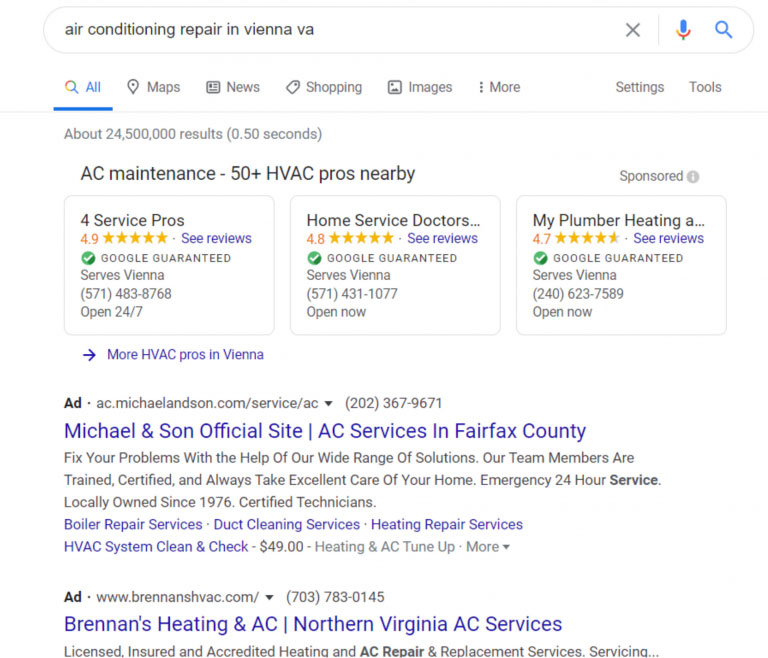The image captures a screenshot of a shopping search page where someone has typed "air conditioning repair in Vienna, VA" into the search text box at the top. The search query is displayed in black text, accompanied by a black 'X' for clearing the text. A blue microphone icon and a blue magnifying glass icon are also positioned adjacent to the search box.

Beneath the search box, there are several tabs including "All" (highlighted with a rainbow-colored magnifying glass), "Maps," "News," "Shopping," "Images," and "More," followed by "Settings" and "Tools." These tabs allow the user to refine the search according to different categories.

The results show a query related to air conditioning repair, with prominently displayed suggestions for AC maintenance services. Three key service providers are highlighted within rectangular boxes:

1. The first box features "Four Service Pros," which has a rating represented by five yellow stars and a blue link reading "See reviews." It is marked with a "Google Guaranteed" badge denoted by a green circle with a white check mark.

2. The second box lists "Home Service Doctors," displaying a rating of 4.8 in red text along with five yellow stars. It also includes a blue link labeled "See reviews."

3. Below these, there is a prompt in blue text and an arrow indicating "More HVAC pros in Vienna."

Additionally, a black "Ad" label is visible, indicating that at least some of the displayed listings might be sponsored advertisements.